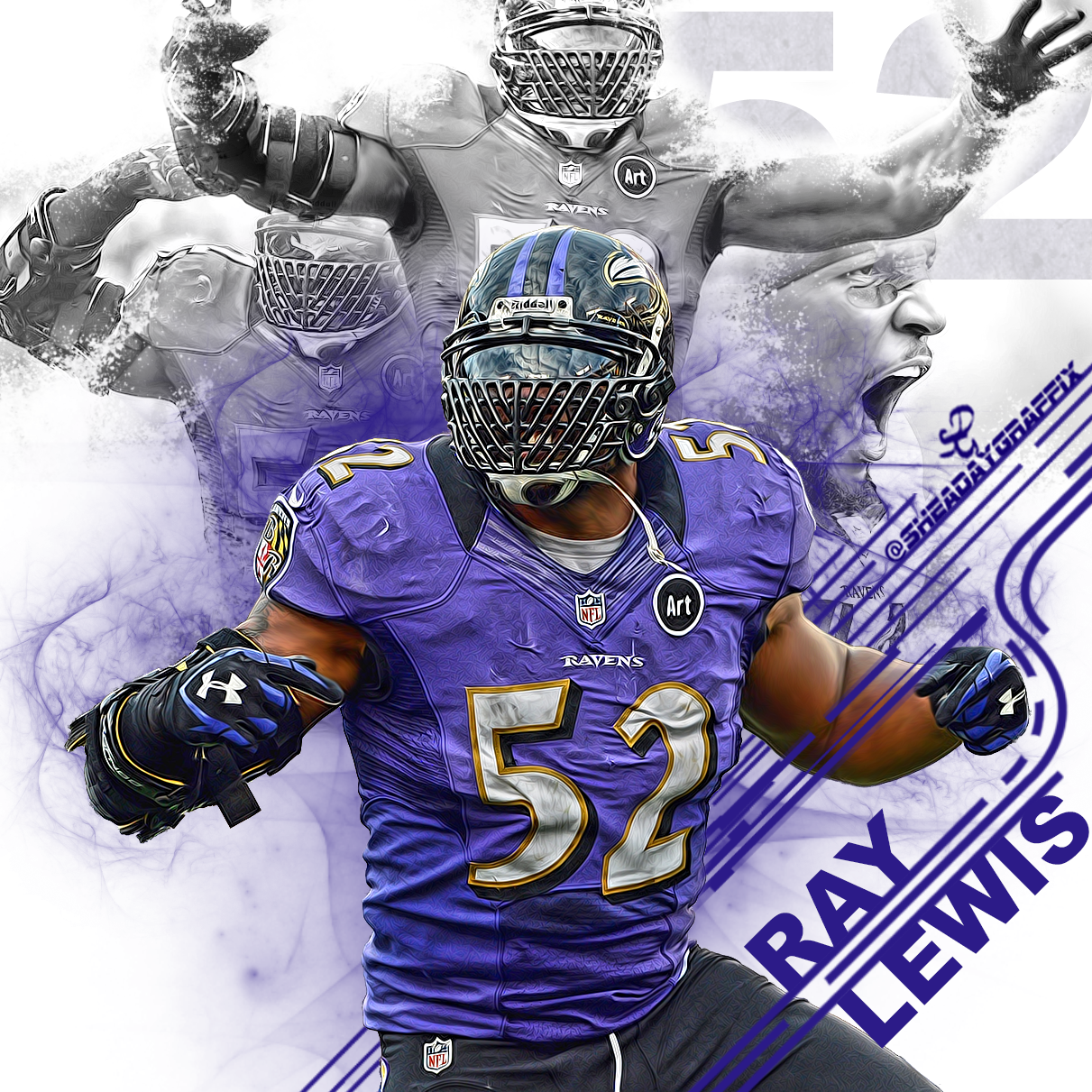The image is a detailed poster of NFL player Ray Lewis, prominently featuring him in a central, full-color photograph. Ray Lewis is wearing a Baltimore Ravens football jersey in purple, with the number 52 in white bordered by yellow both on the front and on his shoulder pads. Underneath his jersey, he has a white shirt, and he pairs this with gray pants. His hands are clad in black gloves adorned with purple stripes. Completing his uniform, he dons a black helmet with purple stripes running down the center, a black face mask equipped with a reflective visor, and a white chin strap. The helmet also showcases a cartoon-styled raven facing forward, characterized by a yellow border, a white beak, and a black head.

In the background, the poster transitions to black and white, displaying various poses of Ray Lewis and a prominent close-up of his face on the right side. Purple text at the bottom right of the full-color image spells out "Ray Lewis." The right side of the image also features a design with purple lines and the name "Shaday Graphics" in matching purple text.